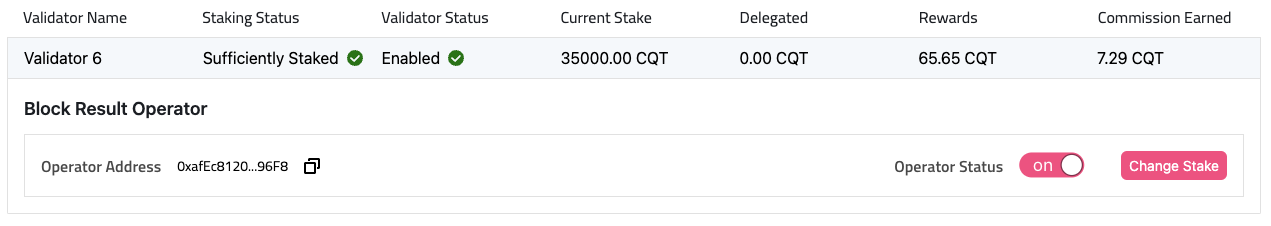This image displays the final section of a multipage document, likely summarizing information from previous pages. The layout is straightforward and easy to navigate. 

- **Validator Name**: Validator 8
- **Staking Status**: Sufficiently staked (indicated by a green check mark)
- **Validator Status**: Enabled (indicated by a green check mark)
- **Current Stake**: 35,000.00 CQT
- **Delegated**: 0.00 CQT
- **Rewards**: 65.65 CQT
- **Commission Earned**: 7.29 CQT
- **Block Result Operator**: Includes the operator address
- **Operator Status**: Displayed in a red box indicating "Off"
- **Change Stake**: Displayed in another red box

The detailed status information ensures clarity regarding the validation process and the operator's current standing.